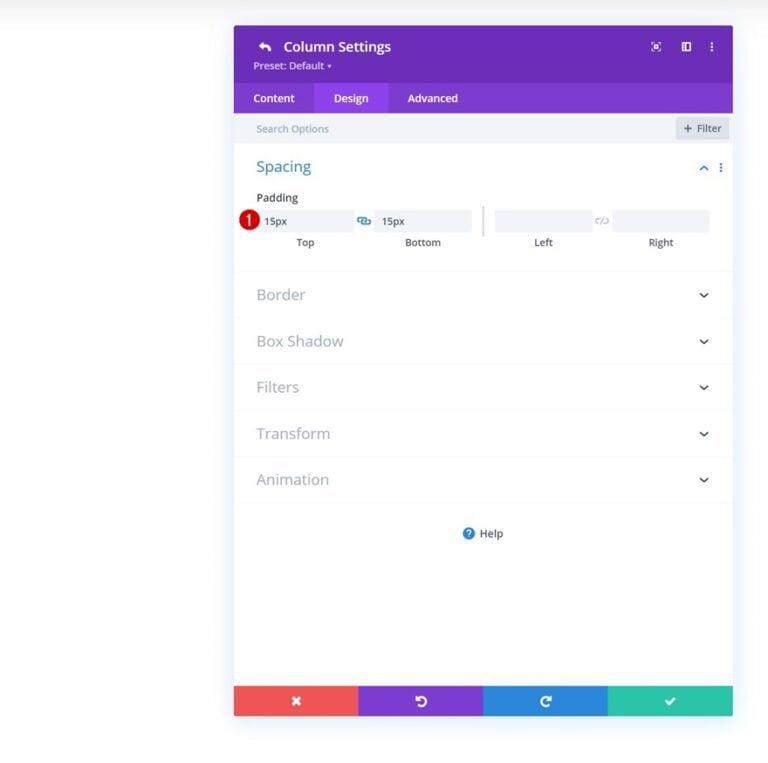This image displays various interface elements likely related to a design or editing software. In the top left corner, there's a left-facing arrow. The main interface appears to be divided into several columns. The first column includes options like "Inch," "Percent," and "Default," with some text indicating the color purple. Below are tabs for "Content," "Design," and "Filter." 

Under the "Advanced Search Options," there are settings for filter and spacing, including a padding range displayed in a red circle stating "1 to 15 pixels," and a chained value set to 15 pixels. 

The interface continues with a gray rectangle indicating "Top" and "Bottom" padding and references to "Left" and "Right" borders. There is a dropdown menu under this section labeled "Border." Below, there are options for "Box Shadows," "Filters," "Transform," "Animation," and a section for "Help."

Additionally, the interface outlines color-coded elements: a red rectangle, a purple rectangle, a blue rectangle, and a green rectangle marked as a checkpoint. These colored shapes appear to be part of the design layout or indicators within the software.